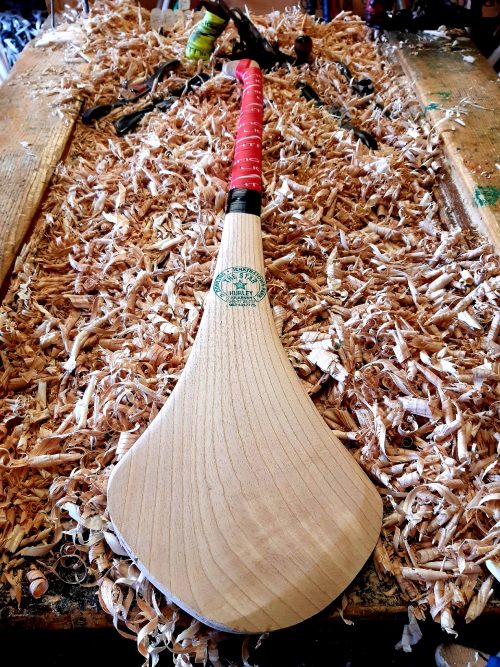The image shows an indoor scene with a rectangular photograph approximately five inches high and three to four inches wide. It depicts a workshop setting viewed from above, focusing on a large amount of beige-brown wood shavings scattered across what appears to be a wooden crate or shelf. In the center of the image lies a prominent, light tan wooden paddle, showcasing its raw wood grain. The paddle features a red strappy handle near the top, transitioning into a thin black wrap at the base where it flares into the wider paddle section. A green circular stamp is visible at the junction of the handle and paddle, possibly reading "Hurley" or "Holly". Two wooden beams, resembling two-by-fours, frame the scene on the left and right sides, acting as boundaries within the crate or shelf. Additionally, partially obscured by wood shavings at the top of the image, a black metal object with a green spherical component is visible, though its exact nature is unclear. The overall composition conveys a cluttered, yet intriguing snapshot of a woodworking space filled with rustic textures and tools.